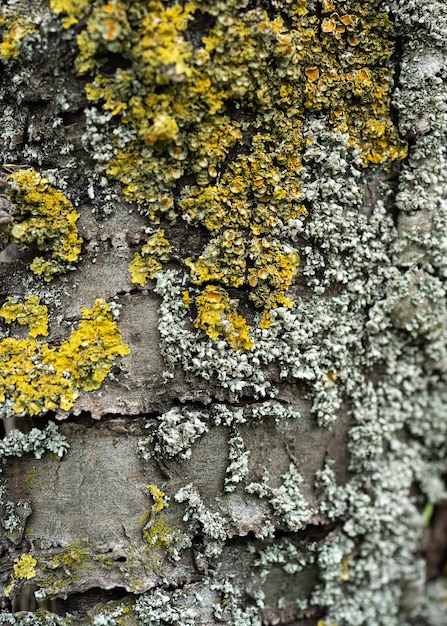This photograph is an extreme close-up of what appears to be the weathered side of a tree trunk, densely covered in various kinds of moss and plant life. The top part of the image is dominated by greenish moss, which transitions into a grayish hue as you move towards the right and bottom sections. The exposed wood beneath is a dry, grayish-brown, adding a sense of aged texture. Here and there, patches of the surface have chipped away, revealing more of the underlying wood. 

The bottom left corner contains a mix of greenish-yellow moss, while the bottom right displays sparse specks of bright green, possibly small stems or new growth. The overall scene seems primarily mossy, accentuated by tiny yellow flecks scattered from the center to the top left, giving the appearance of delicate, shallow growths rather than substantial plants. Additionally, the grayish surface in the background features crevices and cracks, adding depth and a rugged texture to the composition.